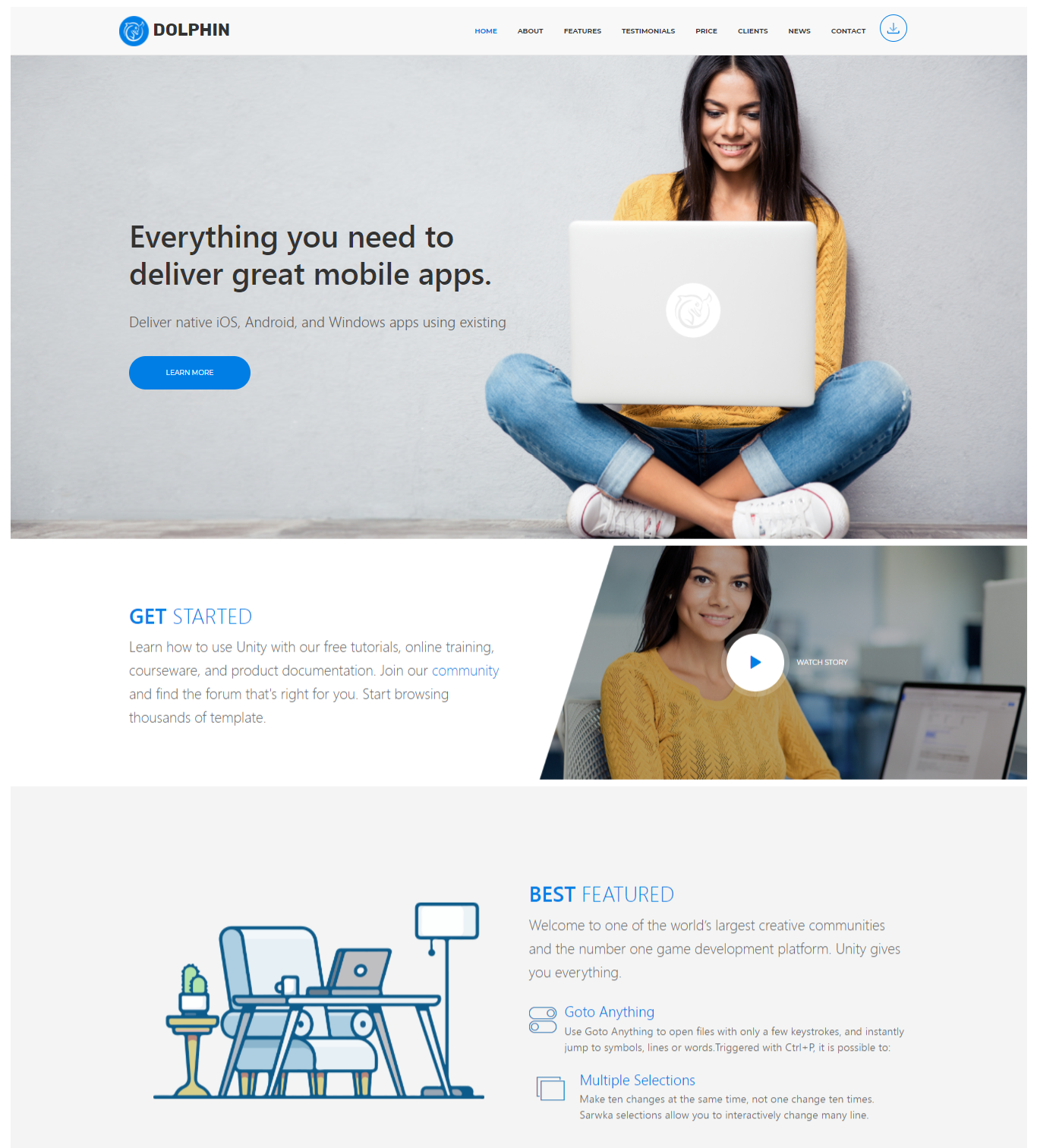This image is a detailed screenshot from a website titled "Dolphin." In the upper left corner, the Dolphin logo is prominently displayed next to a horizontal list of menu items: Home, About, several unreadable items, Price, Clients, Move, and Compact.

Dominating the center of the image is a woman seated on the ground. She is dressed in a yellow sweater and blue rolled-up jeans, paired with white Converse sneakers. A laptop rests on her lap, and her legs are bent and crossed at the ankles. To the left of this central image, text reads: "Everything you need to deliver great mobile apps. Deliver native iOS, Android, and Windows apps using existing." Below this text, there's a blue button labeled "Learn More."

On the right side of the image, a close-up of the same woman is visible from the chest up. She is smiling and looking directly into the camera, with an open laptop beside her. Text beside this image encourages users to "Get Started," offering resources such as free tutorials, online training, courseware, and product documentation. It invites viewers to join the community, find appropriate forums, and start browsing thousands of templates.

Below this, the left side of the image features an animated illustration depicting a cozy armchair accompanied by a desk, laptop, lamp, and a potted plant. Adjacent to this illustration, text proclaims: "Best Featured. Welcome to one of the world's largest creative communities and the number one game development platform. Unity gives you everything." Although some subheadings and selections are too small to read, the overall message highlights the comprehensive offerings and community support available through the platform.